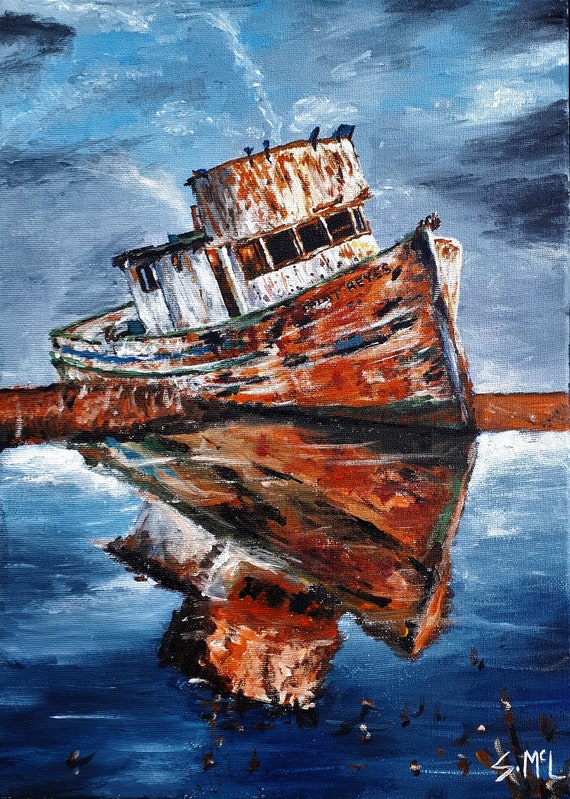This portrait-oriented painting vividly captures a dilapidated white vessel, reminiscent of a rusted fishing crawler, grounded on a sandbar that spans horizontally across the center of the composition. The ship, with its corroded brown and orange edges, is tilted to the left, exposing its underbelly. Broken windows punctuate the front area of the captain's cabin, and a partial name "T. Reyes" is visible on the right side of the hull. The reflective surface of the water below mirrors the damaged vessel, amplifying its state of wreckage. Above looms a dramatic sky, swirling with dark blues, grays, and streaks of white clouds, contributing to the somber atmosphere. Smaller, indistinct specks near the bottom might suggest fish or seabirds, adding to the rustic and desolate aesthetic. In the bottom right corner, the artist’s initials, SMCL, are marked in white, completing this evocative portrayal of maritime decay.